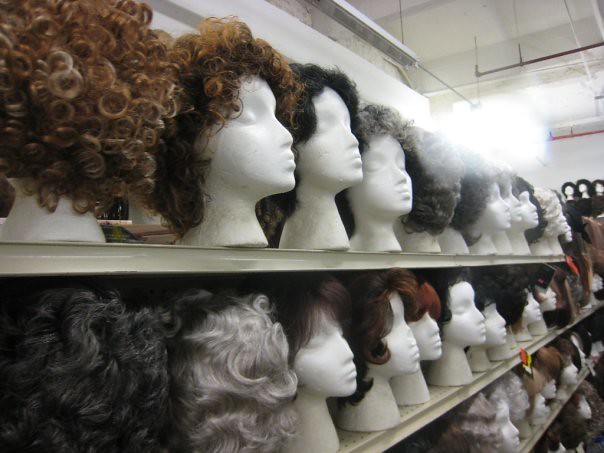This photograph captures a detailed scene inside a wig store, showcasing four long metal shelves filled with a variety of wigs, each placed on Styrofoam mannequin heads. The shelves stretch diagonally from the front left to the back right of the image, creating a perspective where the wigs on the left appear closer. The top shelf features curly brown wigs, with one particularly voluminous wig covering the entire face of its mannequin. Below, the second shelf displays shorter, straight-haired wigs in various shades, including dark brown, light gray, and reddish brown. The following rows present a mix of brown and blonde wigs, with a notable black wavy wig positioned prominently on the bottom shelf. The store has a high, industrial-style ceiling adorned with wires, and a bright light or window glare illuminates the area from the top left corner, enhancing the visibility of the wigs and adding a sense of space. In the background, additional wigs can be seen lining the back wall, further emphasizing the extensive variety available in the store.